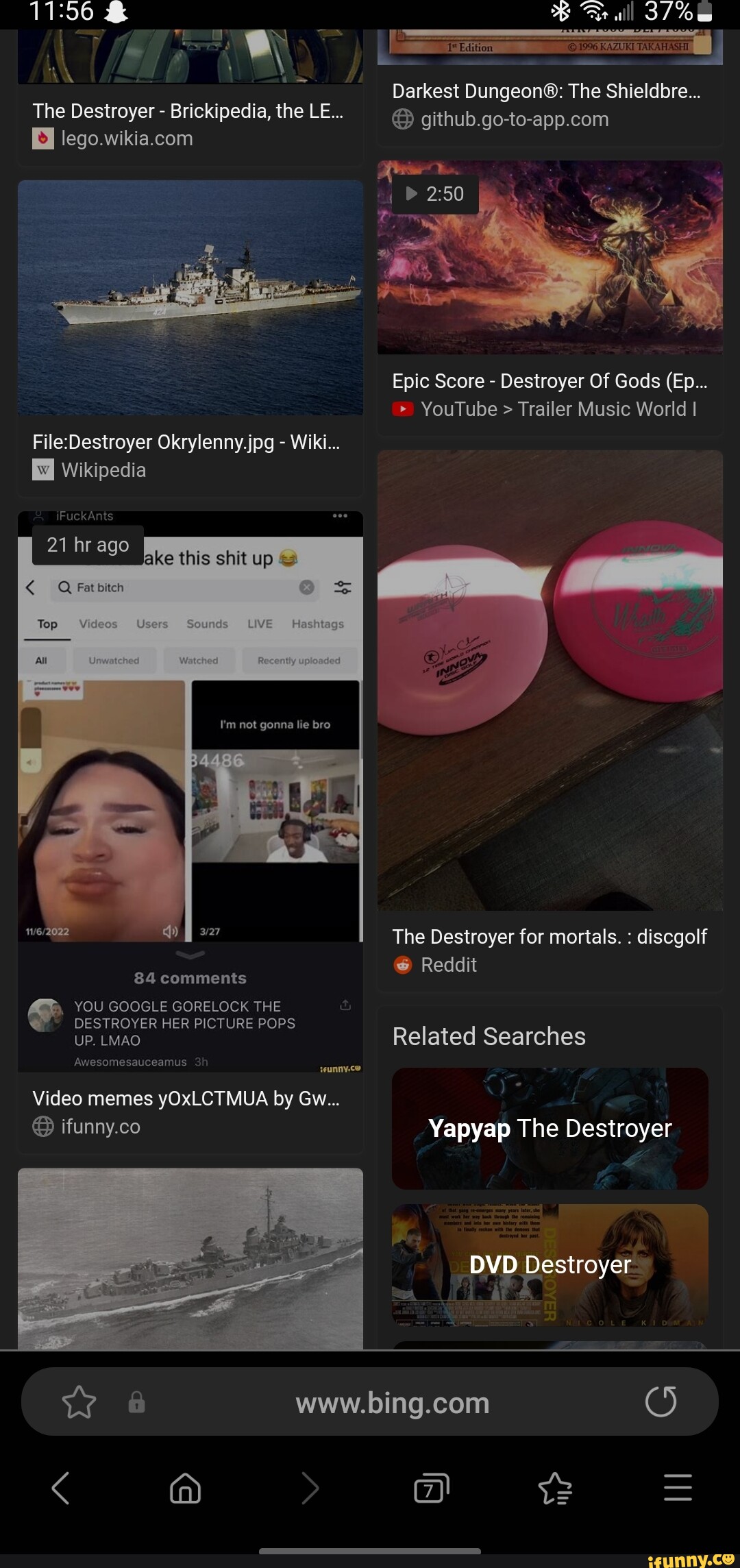This is a screenshot of a Bing search results page featuring various news stories and images. 

Prominently displayed among the results is a photograph of two frisbees—one light pink and one dark pink—lying on a wooden board. A strip of sunlight cuts across these frisbees, creating a striking effect. Below this image is the caption "The Destroyer for Mortals: Disc Golf," sourced from the social media platform Reddit.

Another image in the search results is a photograph of a destroyer ship, captioned "File: Destroyer Oryclenny.jpeg - Wiki," with the source cited as Wikipedia.

Additionally, one of the windows shows a photograph of a woman taking a selfie, with a man appearing to stream from his desk next to her image. The caption above this window reads, "I'm not gonna lie bro."